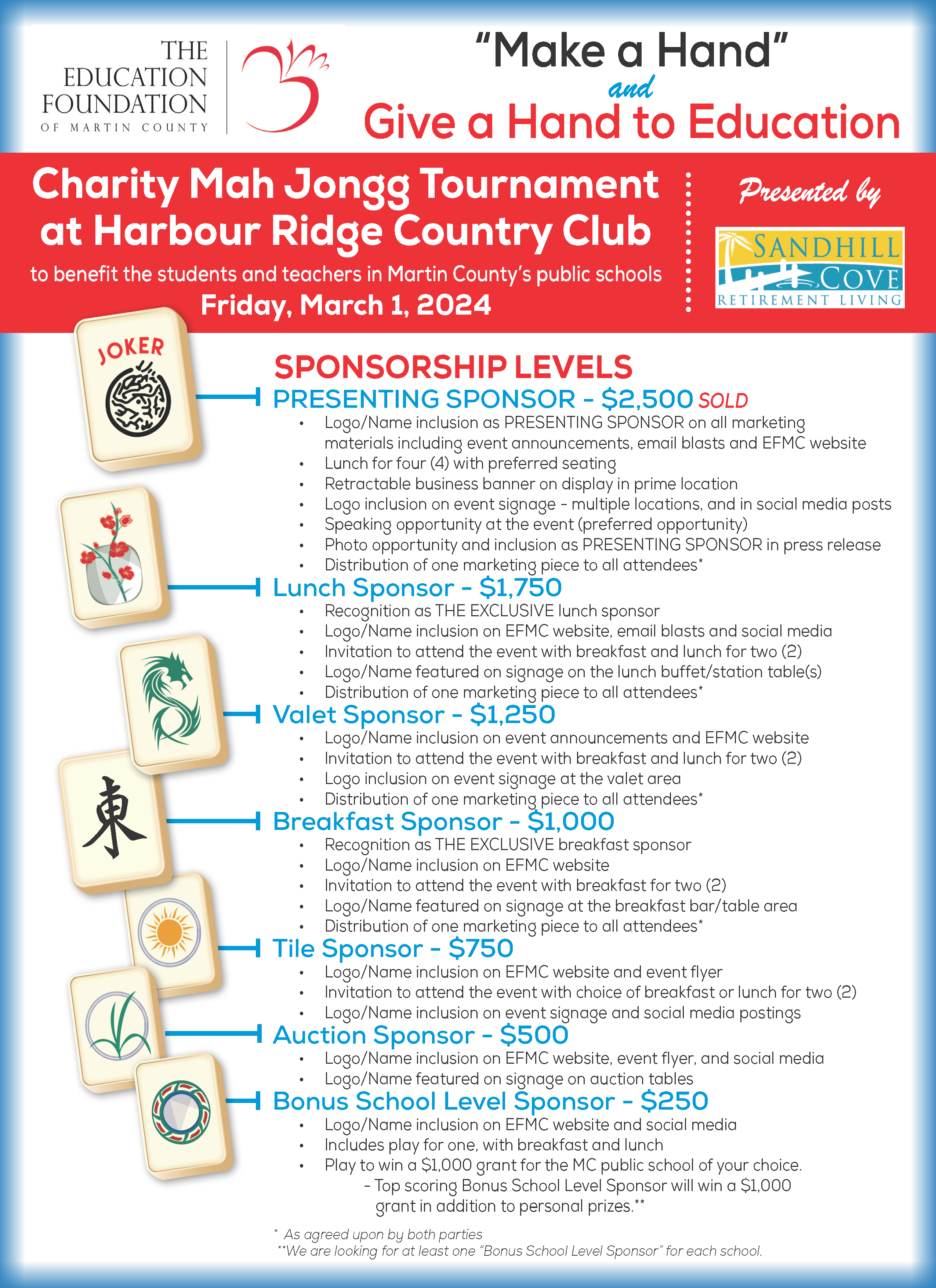This promotional flyer for a charity event, titled "Mahjong Tournament at Harbor Ridge Country Club," is designed to benefit the students and teachers in Martin County's public schools. Organized by the Education Foundation of Martin County and presented by Sand Hill Cove Retirement Living, the event is scheduled for Friday, March 1, 2024. The flyer features a clean white background with a light blue border. In the top left corner, the Education Foundation of Martin County's name appears next to a partial apple logo, while the encouraging slogan, "Make a Hand and Give a Hand to Education," is prominently displayed to the right.

A striking red banner across the top announces the "Charity Mahjong Tournament at Harbor Ridge Country Club," and below, detailed sponsorship levels are laid out. Each sponsorship level is illustrated with a different mahjong tile on the left. The levels are as follows:

1. **Presenting Sponsor** - $2,500 (sold, represented by the Joker tile)
2. **Lunch Sponsor** - $1,750 (represented by a vase tile)
3. **Valet Sponsor** - $1,250 (represented by an S tile)
4. **Breakfast Sponsor** - $1,000
5. **Tile Sponsor** - $750 (represented by a tile with a circle and sun)
6. **Auction Sponsor** - $500 (represented by a tile with a circle and grass)
7. **Bonus School Level Sponsor** - $250 (represented by a tile with an ornate wreath)

This detailed flyer not only highlights the event and its purpose but also provides an elegant and organized breakdown of sponsorship opportunities, each associated with unique mahjong tile imagery, enticing potential sponsors to contribute to the cause.